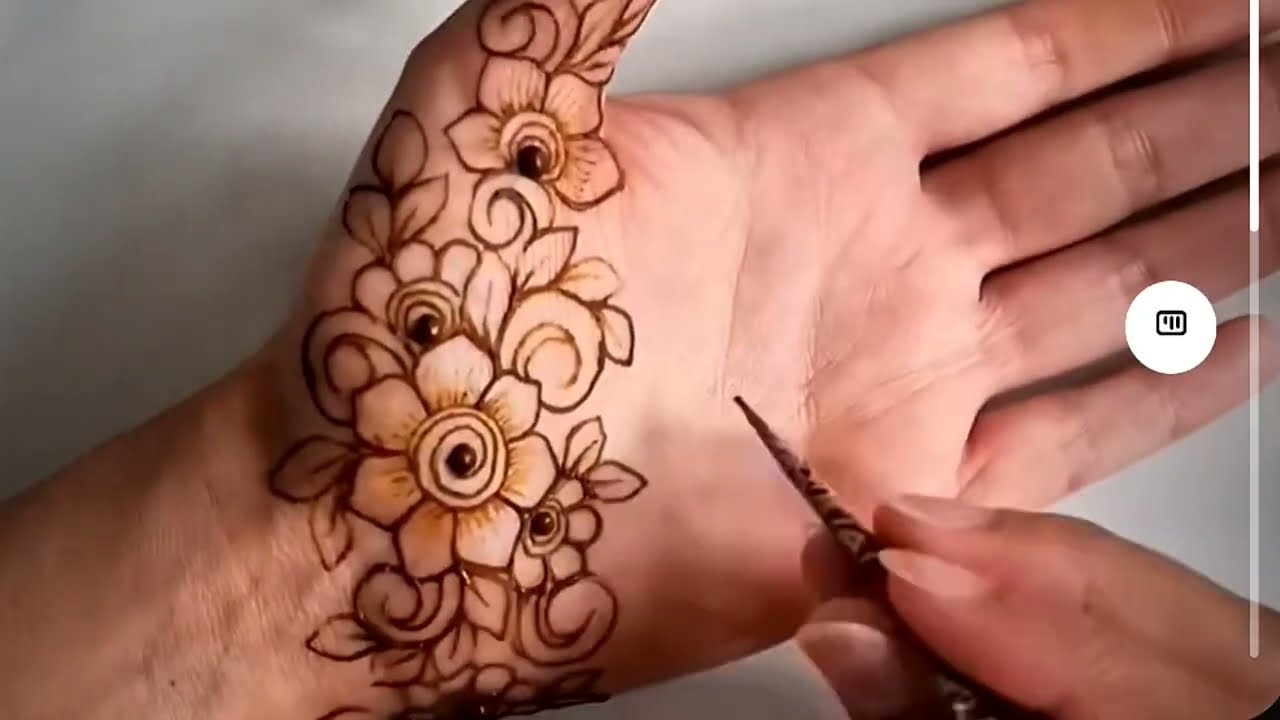In this image, a person's left hand, palm-up, rests on a white surface. The hand, which appears to be Caucasian, is intricately decorated with a detailed flower pattern that extends from the bottom of the palm up to the thumb. The artwork includes various flowers, each with petals encircling a central swirl and black dots. Surrounding these flowers are numerous leaves, filling in any spaces on the skin.

The right hand, holding a brown drawing utensil marked with black ink, appears to be in the process of applying this pattern, suggesting it could be a henna tattoo. The utensil is light brown with a patterned taper towards the tip. The overall scene is set against a white background with a grayish, partially transparent bar running along the right side, hinting at a screenshot from an app. A noticeable button with a black icon featuring three vertical lines is also present within the bar. The composition showcases the intricate floral design and the methodical application of the temporary ink on the hand.